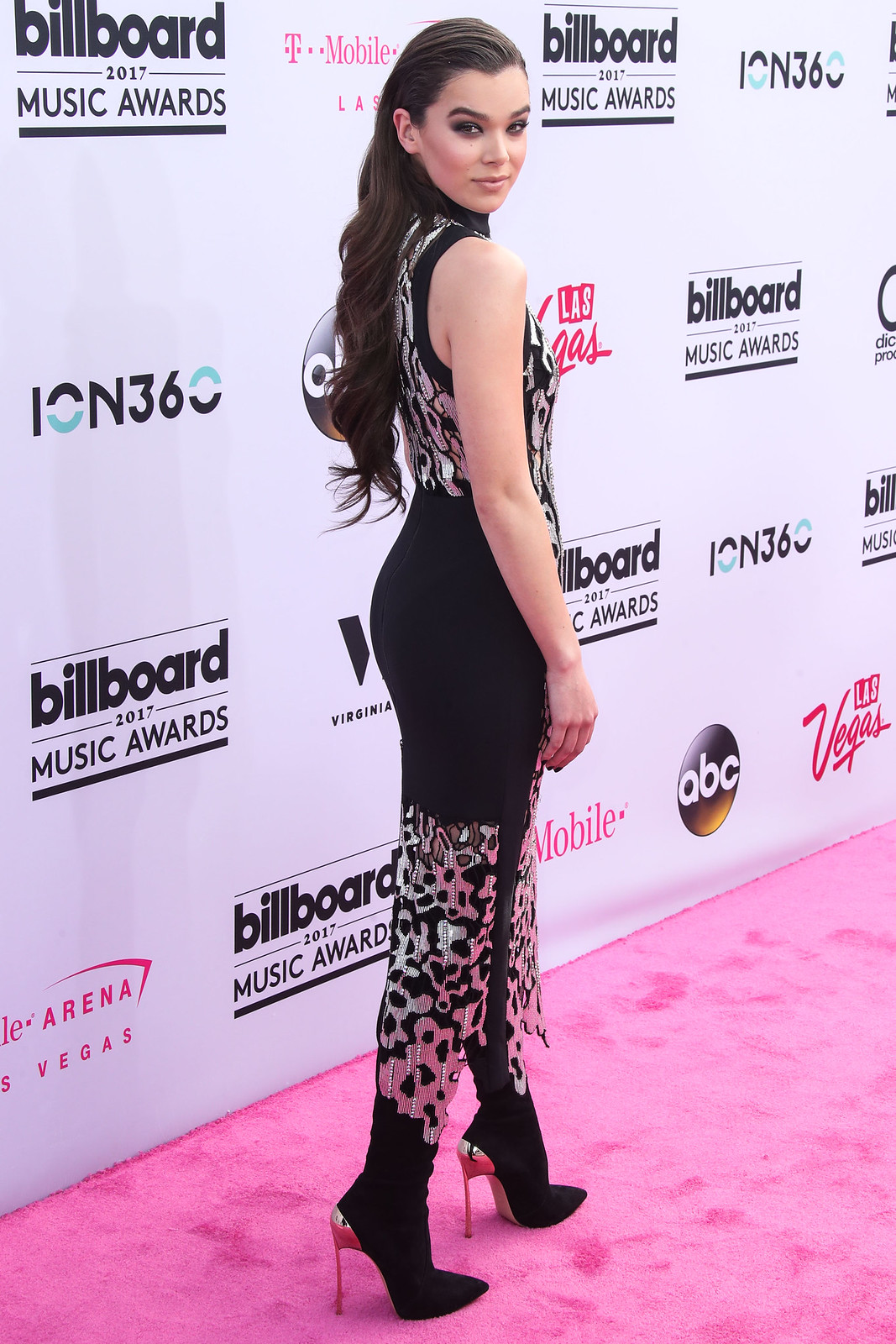This image captures a vibrant scene at the 2017 Billboard Music Awards, set on a strikingly bright fuchsia pink carpet. The backdrop is adorned with an array of logos, including those for the Billboard 2017 Music Awards, Las Vegas, ABC, T-Mobile, and ION 360, all in various colors and fonts, uniformly scattered across the white background. At the center of this lively setting, a youthful celebrity with a light skin tone and long, slightly wavy dark hair poses gracefully. She is dressed in an elegant, sleeveless black gown featuring intricate silver accents that embellish the top, bottom, and front of the dress. Her footwear consists of chic black high-heeled boots with distinctive silver heels. The celebrity, appearing to be in her mid-20s, stands with her body slightly turned away from the camera, her head turned to the right to engage with the lens, and her hand resting gently by her side, creating an effortlessly stylish and poised moment captured on the pink carpet.